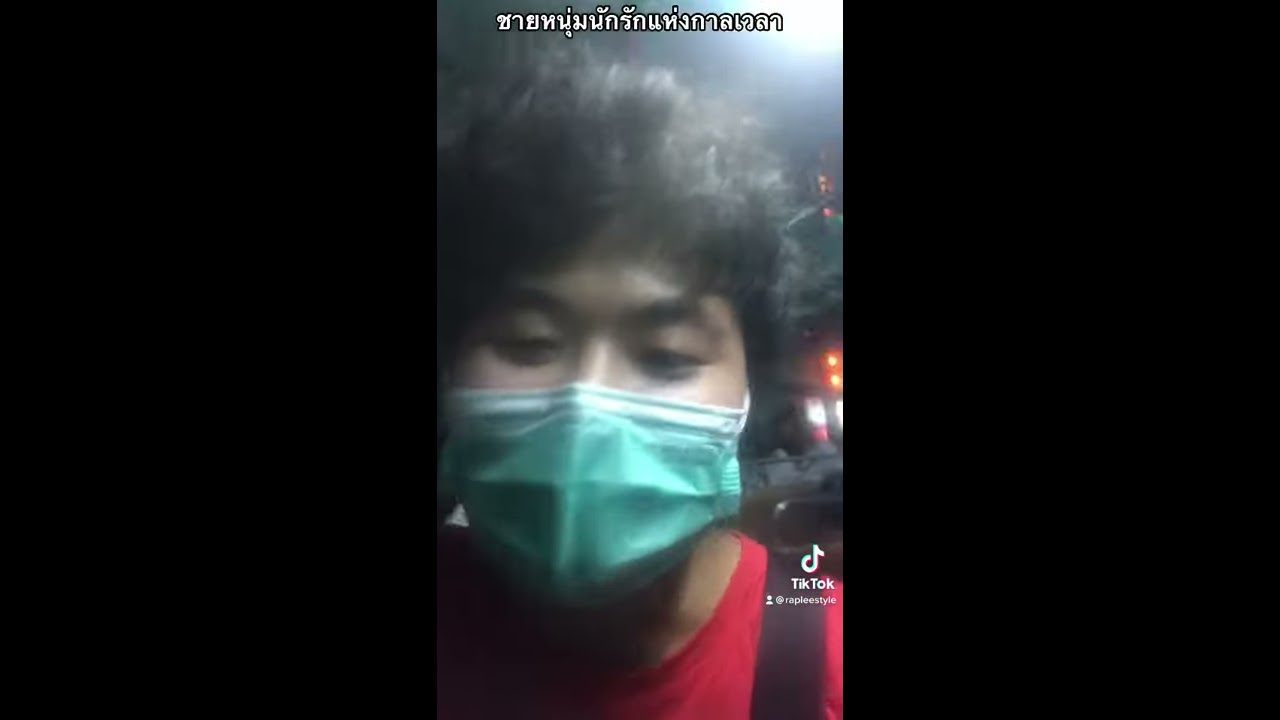In this detailed photographic still from a TikTok video, we see a close-up of an individual of Asian ethnicity, potentially in their 20s, with dark, short, wavy hair and prominent dark eyebrows. The lower half of the face is obscured by a blue and white surgical mask. The individual is wearing a red scoop-neck T-shirt and has a black strap over their left shoulder, suggesting they might be carrying a bag. The image features a horizontal rectangle format with a highlighted vertical rectangle in the center showcasing the person's face from the neck up. The background is likely an indoor public space with harsh, bright white lighting emanating from the upper right corner, causing a glare over the hair. The overall ambiance indicates it might be nighttime. There are people or indications of activity in the distant background. White text in a non-English language appears at the top of the image, contributing to its distinct cultural context. Additionally, there is a TikTok logo towards the bottom right corner of the highlighted part, with the text "TikTok Rapley style" inscribed below it. The image has wide black borders on the left and right sides.